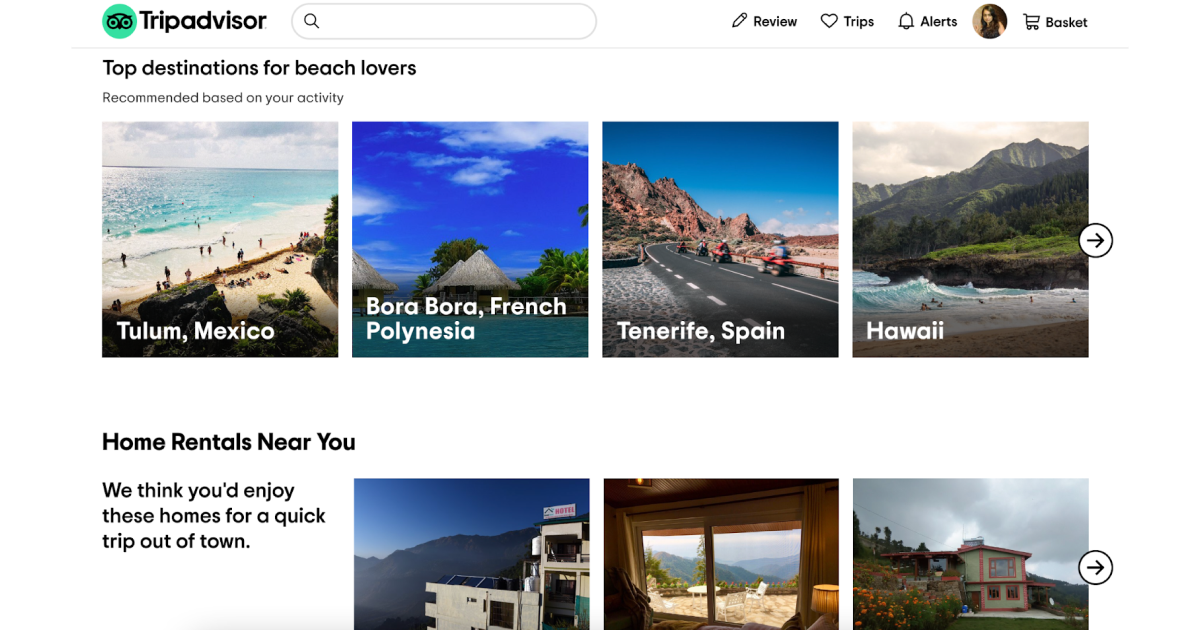The image is a screenshot of the TripAdvisor homepage. Dominating the top left is the TripAdvisor logo, characterized by a green owl with large, expressive eyes. To the right of the logo are several elements: 

- A search bar for locating hotels, destinations, and more.
- A pencil icon indicating the option to write a review.
- A heart symbol representing 'Trips.'
- A bell icon for alerts.

A user is currently logged in, represented by a profile picture of a woman appearing to be in her 20s.

Below the TripAdvisor logo, in slightly smaller text, the header "Top Destinations for Beach Lovers" is displayed. This section showcases four exotic destinations, each paired with an eye-catching image:

1. **Mexico:** A bustling coastal scene filled with people enjoying the seaside.
2. **Bora Bora, French Polynesia:** A breathtaking view featuring mountains and a blue sky dotted with clouds.
3. **Tenerife, Spain:** Adventurers riding ATVs in a scenic locale.
4. **Hawaii:** Majestic volcanoes and inviting ocean waves.

Further down the page is a section titled "Home Rentals Near You," suggesting accommodations for brief getaways. A description accompanies this section, which features three images of home rentals. Each section has arrows for users to expand and view more options, both for beach destinations and nearby home rentals.